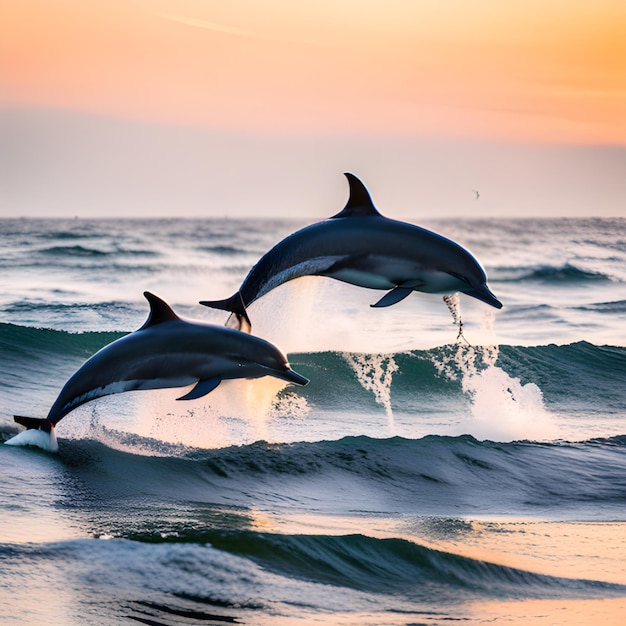This photograph captures two gray dolphins leaping out of a choppy ocean, with water droplets splashing off their sleek bodies as they soar in midair. Below them, four distinct waves ripple across the water's surface. The dolphin positioned higher in the air is slightly behind and larger than the one in the front, which is smaller and closer to the viewer. The backdrop features an expansive, orange-hued sky, blending from a vibrant yellow near the horizon to a purplish tint above, suggesting either dawn or dusk. A silhouetted bird, likely a seagull, can be seen flying in the distance, and an indistinct landmass or mountainous terrain lies on the horizon, adding depth to the serene yet dynamic scene.